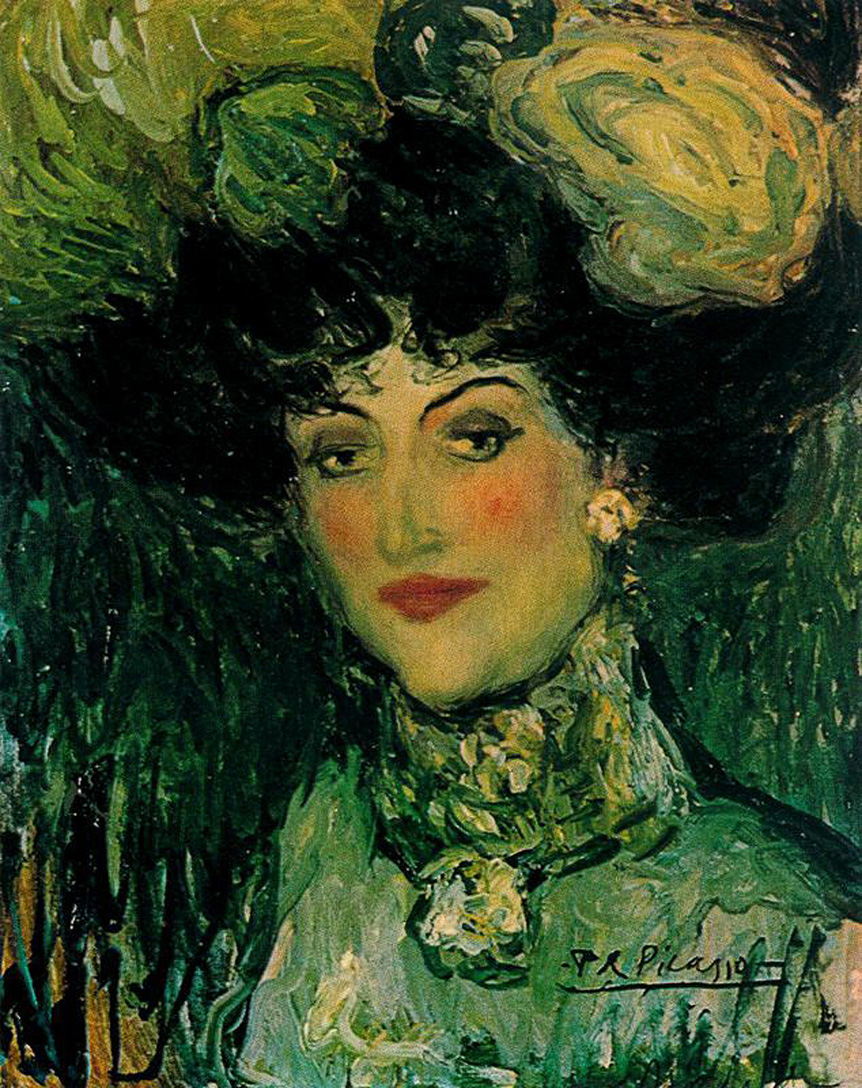This oil painting, slightly impressionist in style, portrays a woman with dark, possibly black hair, adorned with a large, decorative hat that extends beyond the top edge of the canvas. Her face and upper body dominate the composition, rendered with bold, chunky brushstrokes, particularly in the background and parts of her clothing. She wears a green top with a high, thick collar reaching up to her chin, complemented by white, flowery earrings. Her pale skin is accentuated by heavy makeup, featuring pronounced blush on her cheeks and bright red lipstick, along with high-arched eyebrows. The background is a vibrant green, interspersed with darker greens and some brown and black strokes on the left side, and lighter green hues around the shoulders. The bottom-right corner of the painting bears an underlined, cursive signature that appears to be "P.R. Picasso," indicating the artist's name.